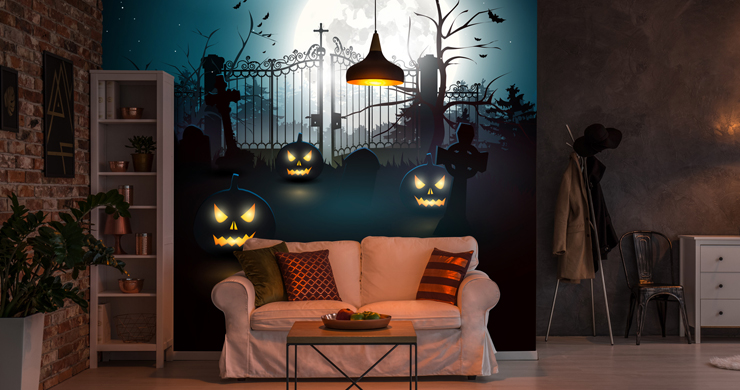The image showcases a horizontal-rectangular photograph of a living room with a distinct Halloween theme. At the center of the room, there's a white loveseat adorned with striking red, orange, and black pillows. In front of the sofa stands a table with a tray of fruit. The background is dominated by an expansive Halloween-themed mural depicting a cemetery gate, a nighttime scene with a large moon, jack-o'-lanterns, tombstones, bats, and roosting birds, lending a spooky atmosphere to the entire room. Flanking this scene on the left side is a white cabinet filled with various objects, including copper items, and a brick wall. On the right side, there's a black chair, a white dresser, and a rack with a jacket hanging from it. Suspended around the room are three jack-o'-lanterns, further enhancing the eerie, festive ambiance. Beyond the sofa, tall wrought-iron gates are visible, giving the illusion of an outdoor setting just beyond a large picture window.